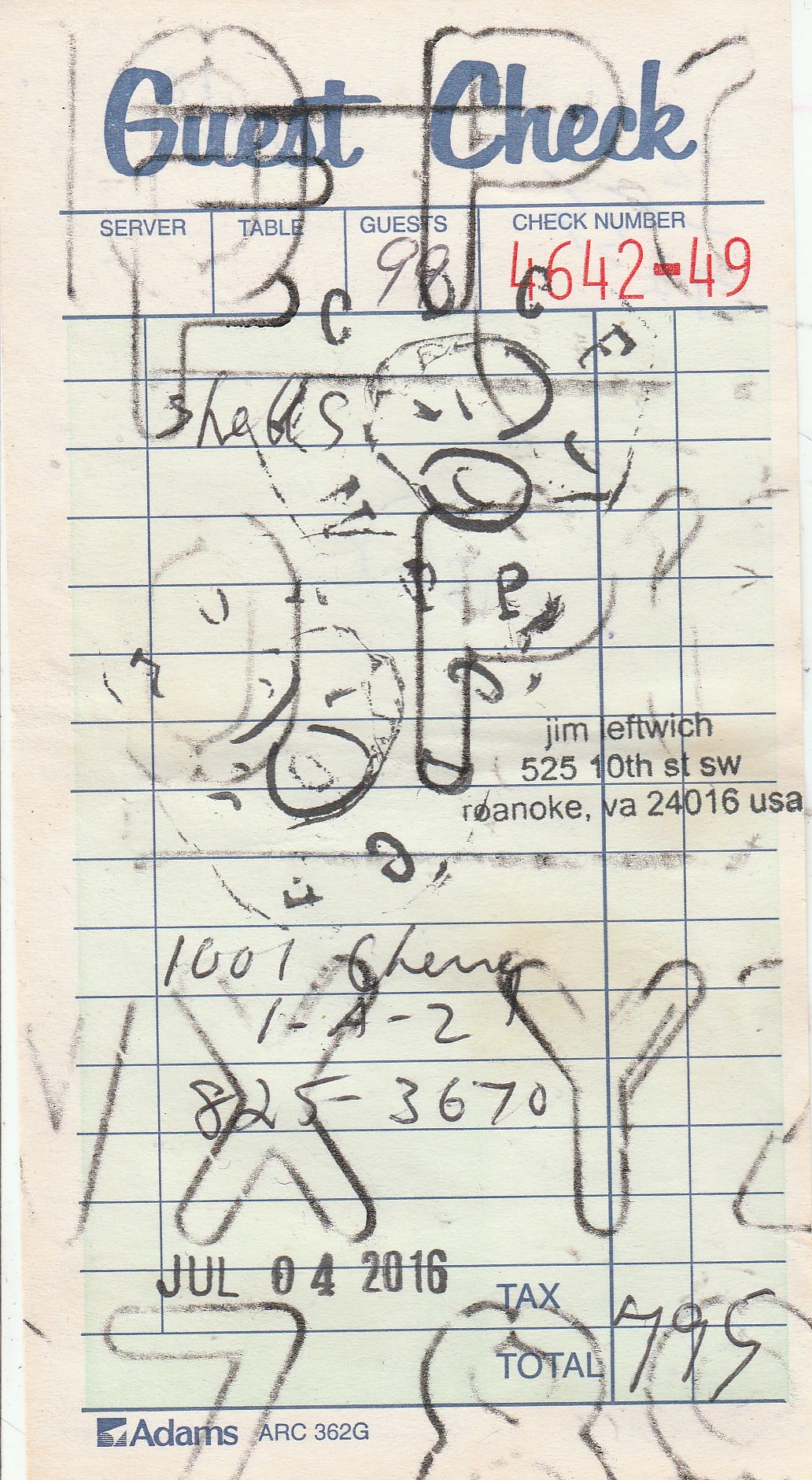This image depicts a detailed guest check similar to those found in diners, featuring a cream-colored top with "Guest Check" written in blue cursive and a light greenish body. Below the header, fields for server info, table details, number of guests, and the check number are outlined. Notably, "guests: 98" and "check number: 4642-49" are inscribed. It appears the check wasn't used for an actual order but contains various notes and stamps. A date stamp reads "July 4, 2016," and prominently displayed is an address: "Jim Leftwich, 525 10th Street Southwest, Roanoke, Virginia, 24016 USA." Additionally, large capital letters, seemingly stamped in black ink as if a child was playing, can be found scattered across the check along with the letters 'X,' 'Y,' and 'P' visible in different areas. There's also a numeric annotation "$7.95" in the total section. Some imprinted letters suggest that another document might have been placed over it for carbon copying. Another text includes "1001 Cherry 1-A-2" and "825-8670."